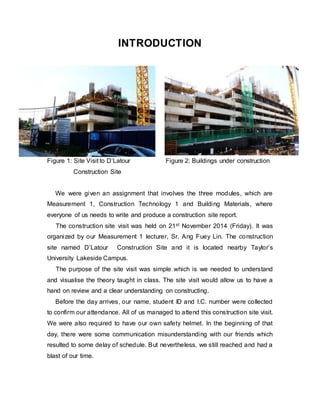This image seems to be an excerpt from a book or research paper, likely an assignment report. The page is predominantly white with a black header at the top reading "Introduction." Below, there are two labeled images. On the left, "Figure 1" depicts a construction site featuring a partially built structure, fences, and construction equipment, including a yellow crane. On the right, "Figure 2" shows what seems to be the same building from a different angle, further along in the construction process, again surrounded by scaffolding and construction materials. Beneath the images, the text explains that the assignment involves three modules: Measurement 1, Construction Technology 1, and Building Materials. The site visit took place on November 21, 2014, organized by the Measurement 1 lecturer, Sir Ang-Fui Lin, at the D. Labor Construction Site near Taylor's University Lakeside Campus. The visit aimed to help students visualize and understand the theory taught in class through hands-on experience. Students were required to wear safety helmets and their attendance was confirmed in advance. Despite some initial communication mishaps, resulting in a delayed start, the visit was ultimately a successful and enjoyable learning experience for all attendees.